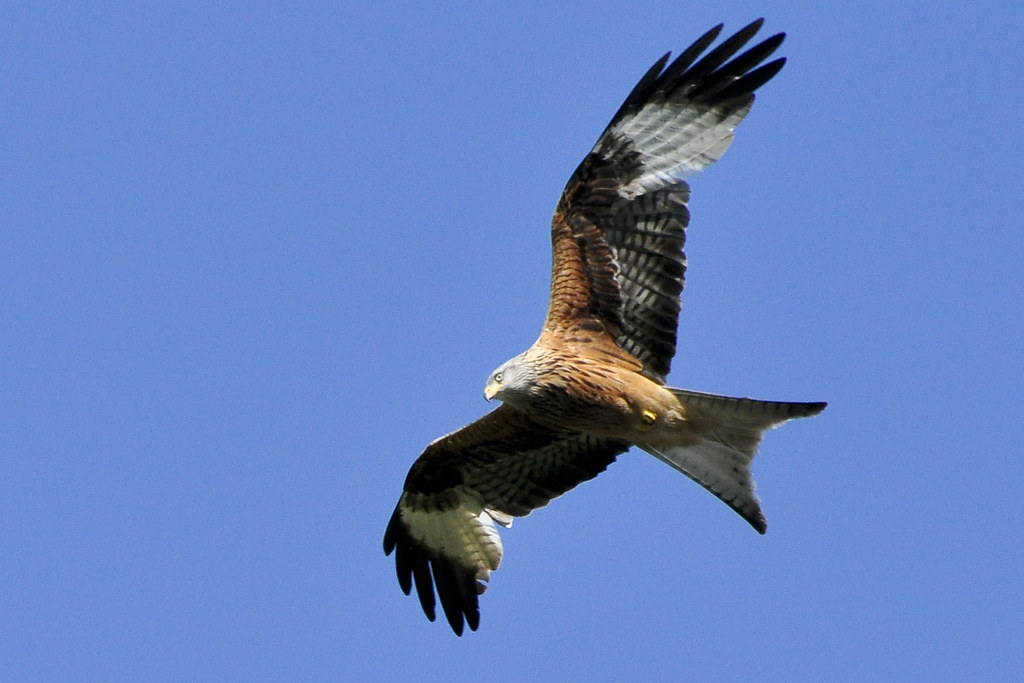This color photograph captures the majestic sight of a large bird of prey, predominantly a hawk or falcon, in mid-flight with its wings magnificently spread against a clear, blue midday sky. Shot from below, the image provides a close-up view of the bird's detailed underbelly and expansive wingspan. The bird showcases a stunning array of feather colors, including shades of white, gray, black, and light brown. The sunlight, casting from the left side, highlights the intricate color variations of its feathers. Notably, the bird features a sharp, pointed yellow beak and small feet tucked neatly against its belly. Its underbelly is predominantly light brown, the tail feathers exhibit a mix of gray and black tips, and the wings transition from brown near the shoulders to black and white further out, adorned with a striking band of white near the edges. The bird’s head appears slightly gray, and the pose suggests a sense of graceful power as it soars through the sky, making this a beautifully detailed and captivating photograph.